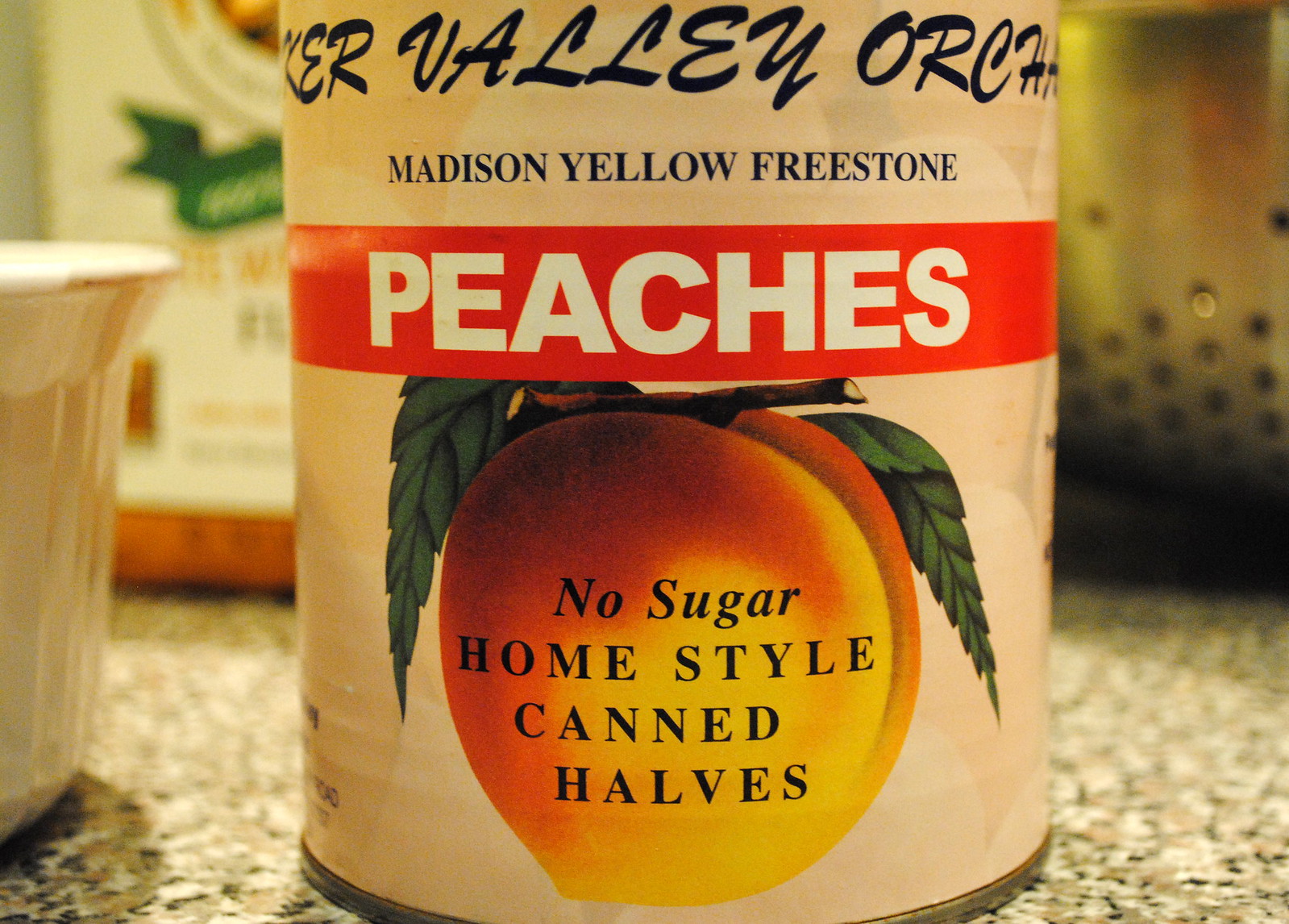The photograph features a can labeled "Valley Orchard Madison Yellow Freestone Peaches" prominently displayed on a granite countertop that is a mix of white, black, and peachy tones. The can has a white background with a bold red band across the middle, adorned with the word "PEACHES" in large white capital letters. Below the red band is a detailed illustration of a peach attached to a branch with leaves, under which the text "No Sugar, Homestyle Canned Halves" is written in black. The brand name "Valley Orchard" is displayed in black, cursive-like capital letters, though part of it is cut off. A light beige vase or cup is situated to the left side of the can. In the blurred background, there appears to be another can or jar with orange and green packaging. Additionally, a metallic sieve is visible in the upper right corner, reflecting part of the peach can. The entire arrangement gives a professional, magazine-like quality to the image.